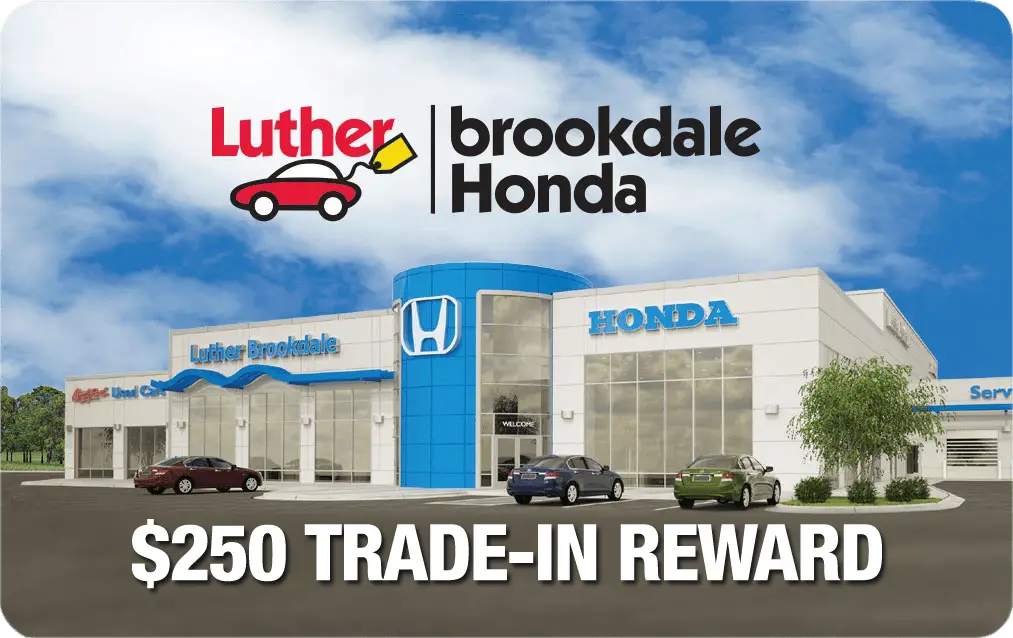The image is a commercial advertisement for Luther Brookdale Honda against a partially cloudy blue sky. At the top of the image, in red text, it reads “Luther,” accompanied by an illustration of a car with a price tag. To the right of this, "Brookdale Honda" is displayed. The main part of the photo showcases the dealership building, which has a distinctive rotunda in the center adorned with a white Honda logo. The building is predominantly white with blue trim, and the name "Honda" is displayed in large blue letters on the right side. Below, in bold all-capital white text, the ad highlights a "$250 trade-in reward." In front of the dealership, three different Honda sedans are parked—a maroon one on the left, a dark blue one, and a green one on the right. The foreground features one tree and four bushes. The service department is visible on the far right.